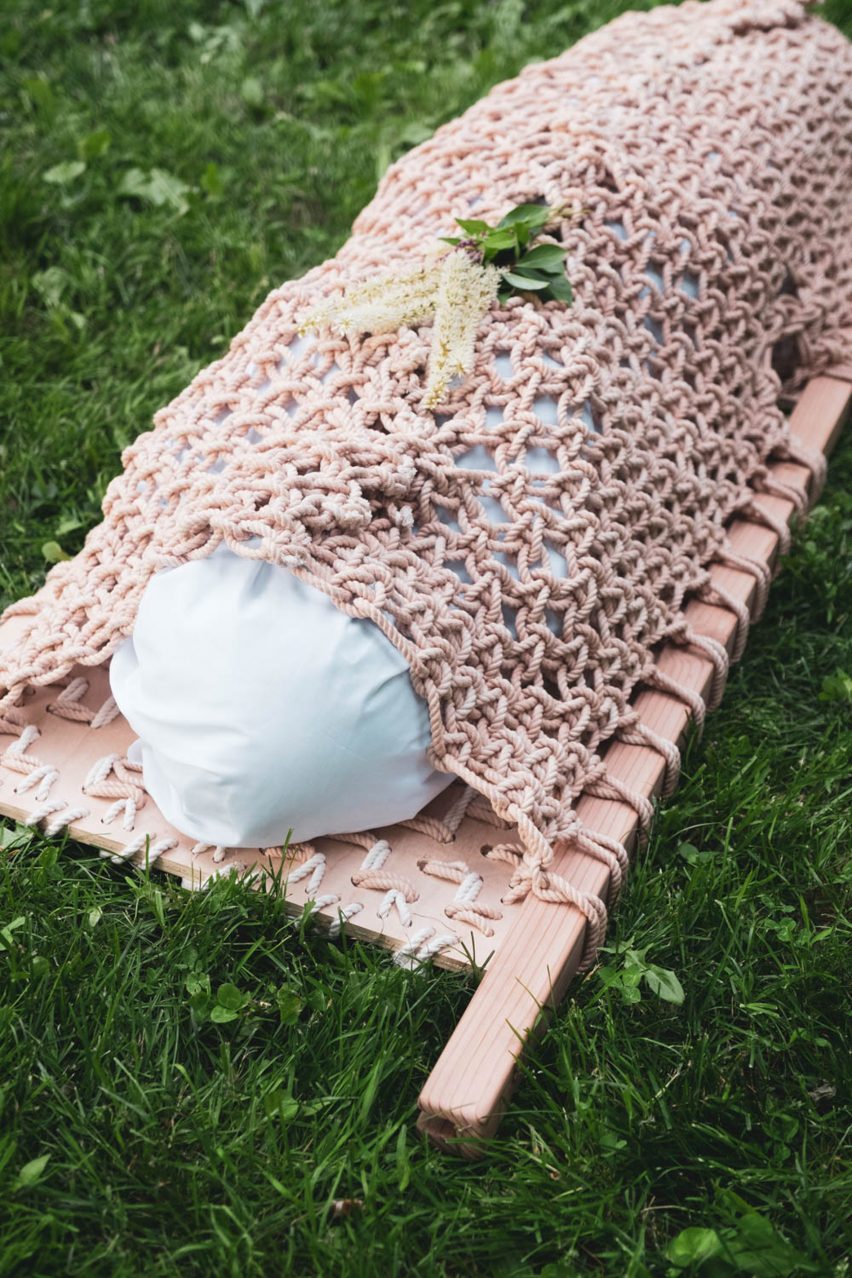The full-color photograph, captured outdoors during the day using natural light, features a vertically rectangular scene set on green grass covering the bottom right, left, and upper left corner. At the center of the image is a handcrafted wooden gurney, constructed with light brown wood and square dowels forming a frame. The gurney has handles on each side, making it easily portable. Across the gurney is a crocheted or knitted beige mesh, securing a white fabric that appears to envelop an object resembling a body. This bundle is placed in a pocket-like section created by the netting. On top of the mesh, there are leaves and white flowers, adding a ceremonial touch to the scene. The overall imagery and accompanying elements suggest a somber, possibly burial-related context.